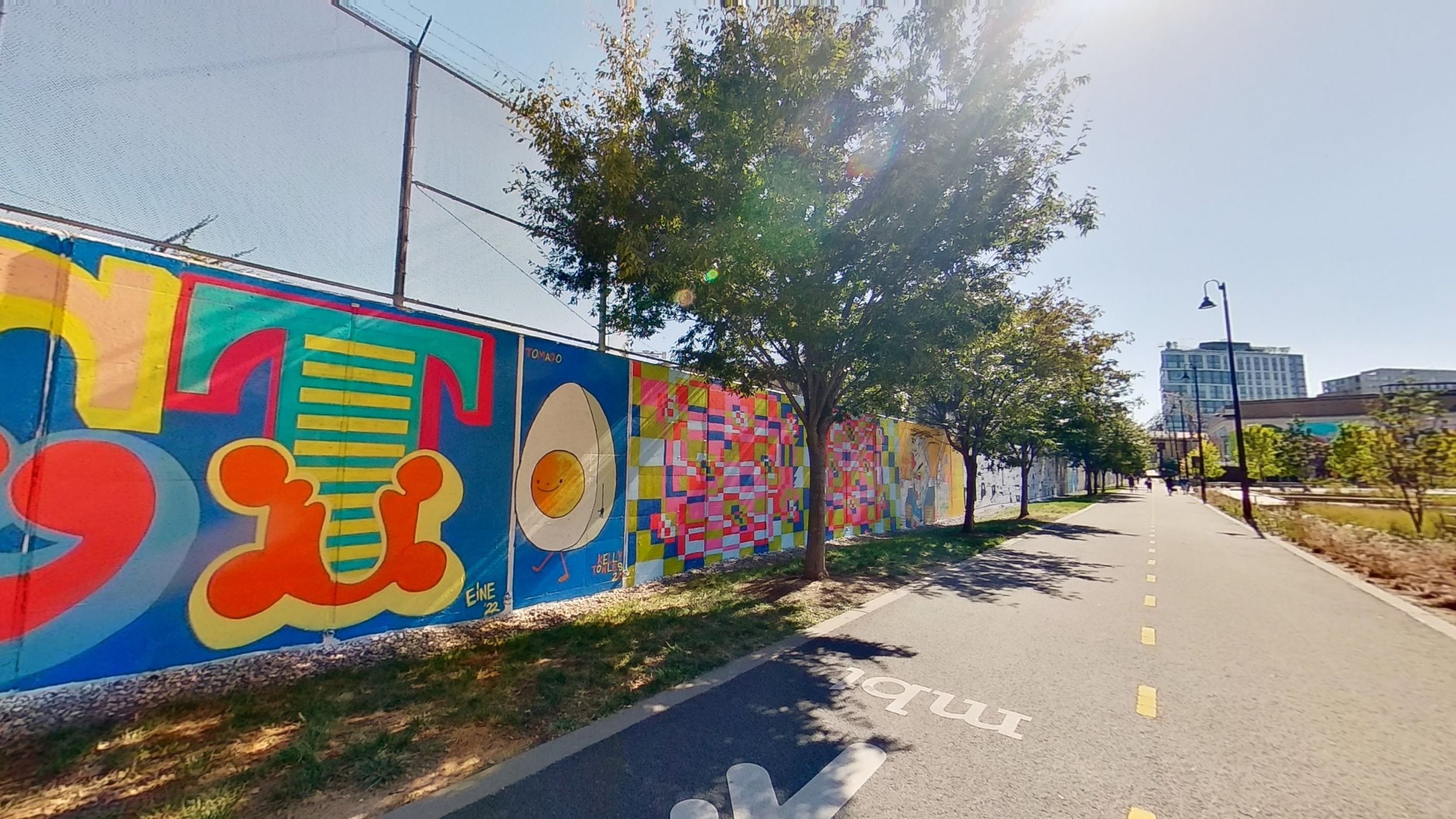The image captures a broad street extending from the bottom left of the frame to the upper right, featuring a central blacktop surface intersected by yellow and white lines, with a visible arrow pointing forward. To the right of the street lies a narrow strip of grass and trees with dense, green foliage and small brown trunks. In the far distance on the right side, there is a rectangular building, approximately ten stories high.

To the left side of the image, there's a long concrete wall adorned with a series of murals. The first mural, closest to the viewer, features a blue background with multicolored letters spelling out "GT" and a depiction of an avocado. Following this, there's a mural of a boiled egg sliced in half, displaying a smiley face on the yolk. Further down, an abstract mural composed of various colored squares, mainly pink, blue, yellow, and white, is visible. Although partially obscured by distance, there appears to be additional artwork, including a smaller piece depicting a person with a hand against their face.

In front of the wall lies a narrow, uneven grassy area mixed with patches of dirt and sand. A chain-link fence topped with barbed wire runs along the top of the wall, adorned with banners featuring blue backgrounds. Above everything, a clear blue sky stretches across the background, while buildings can be seen in the distance on the right.